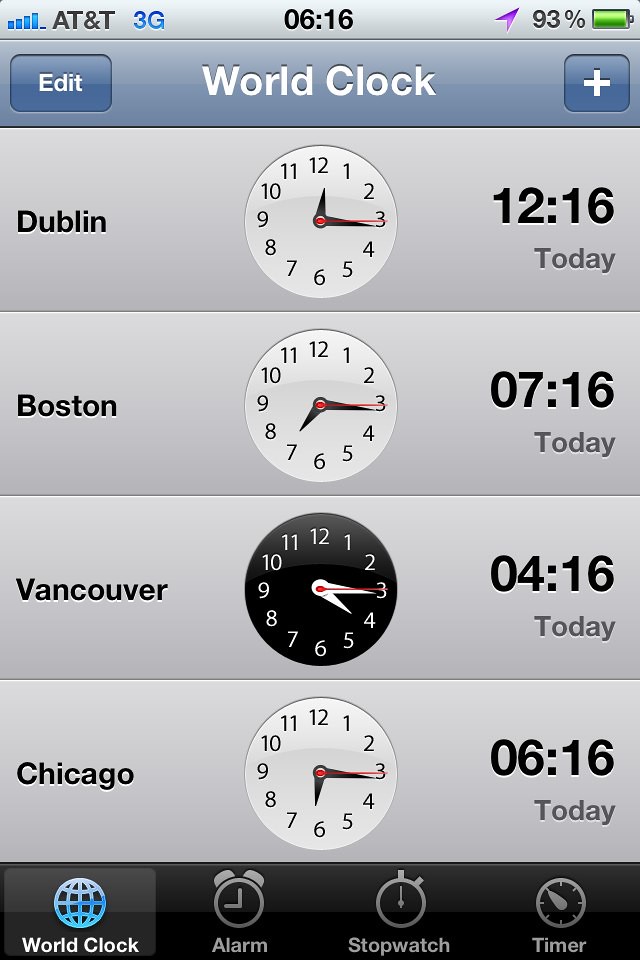The image depicts a screenshot from an iPhone displaying a world clock interface, reminiscent of the older iPhone models around the era of the iPod Touch. At the top left of the screen, the status bar shows "AT&T 3G," with signal strength bars, and at the center, the time is indicated as "06:16." On the right side, there's a location services icon in purple, followed by a "93%" battery level with a green battery icon. Below this, the interface features a headline "World Clock" centered at the top with an "Edit" button on the left and a "+" button on the right. The list of cities includes:

- Dublin with a white clock face indicating "12:16" today.
- Boston with a white clock face showing "07:16" today.
- Vancouver with a black clock face displaying "04:16" today.
- Chicago with a white clock face reading "06:16" today.

At the bottom of the screen, there is a black navigation bar with options labeled "World Clock," "Alarm," "Stopwatch," and "Timer." The detailed arrangement and the color-coded clocks for each city provide a clear and intuitive visualization of different time zones on the iPhone's world clock feature.